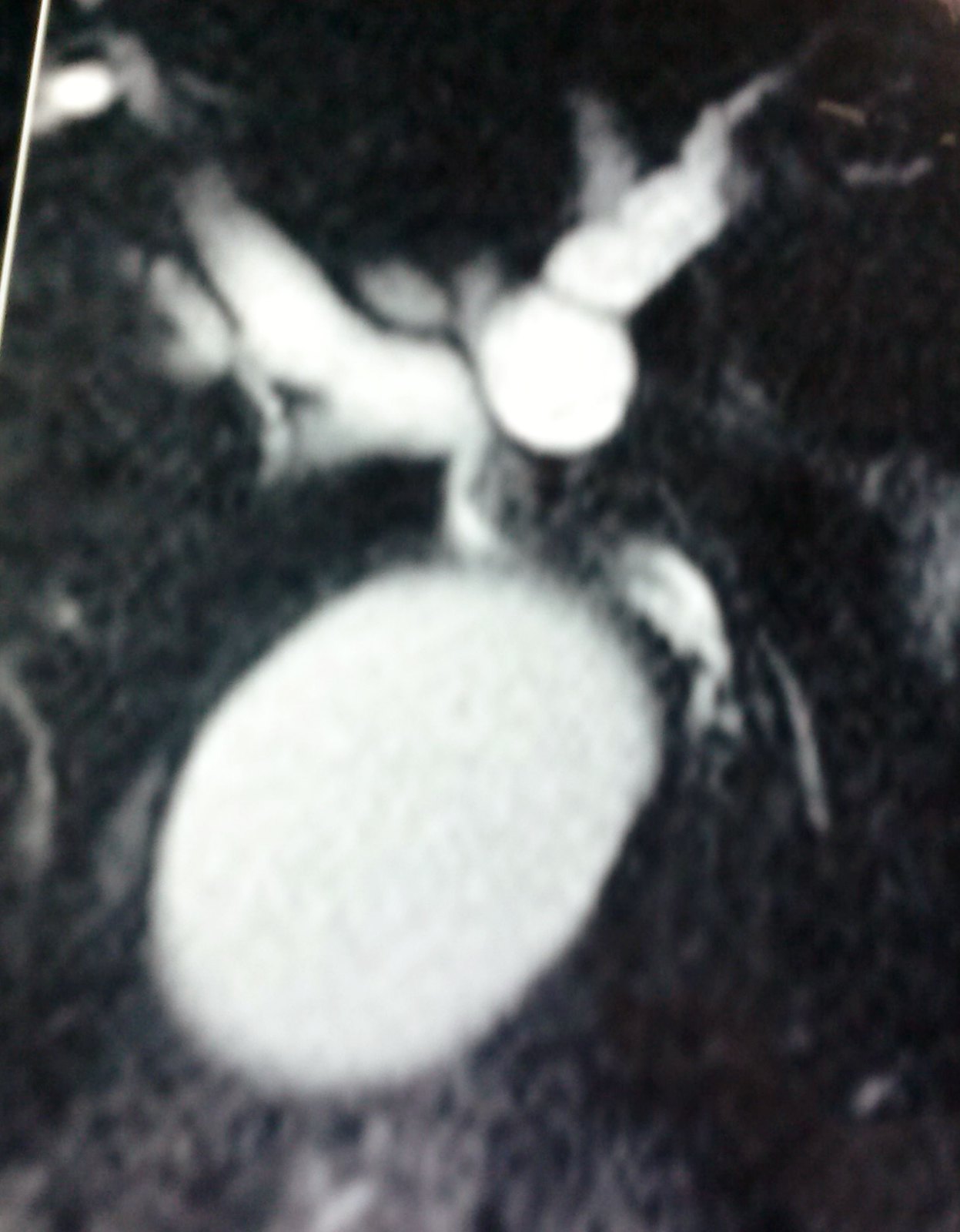This is a blurred, black and white photograph that appears to be a close-up of an unidentified object. Dominating the center of the image is a large, oval-shaped white form, which could be interpreted as an insect or a part of an organism viewed under a microscope, though the actual subject remains ambiguous. Surrounding this central shape are several other white blobs and lines set against a very dark, almost black background. The photograph lacks any identifying text, dates, or colors other than shades of black, white, and gray. The entire composition seems to focus on these abstract forms, with the central white object being the key feature, creating a mysterious and enigmatic visual impression. The image is relatively small, estimated to be around four by six inches.